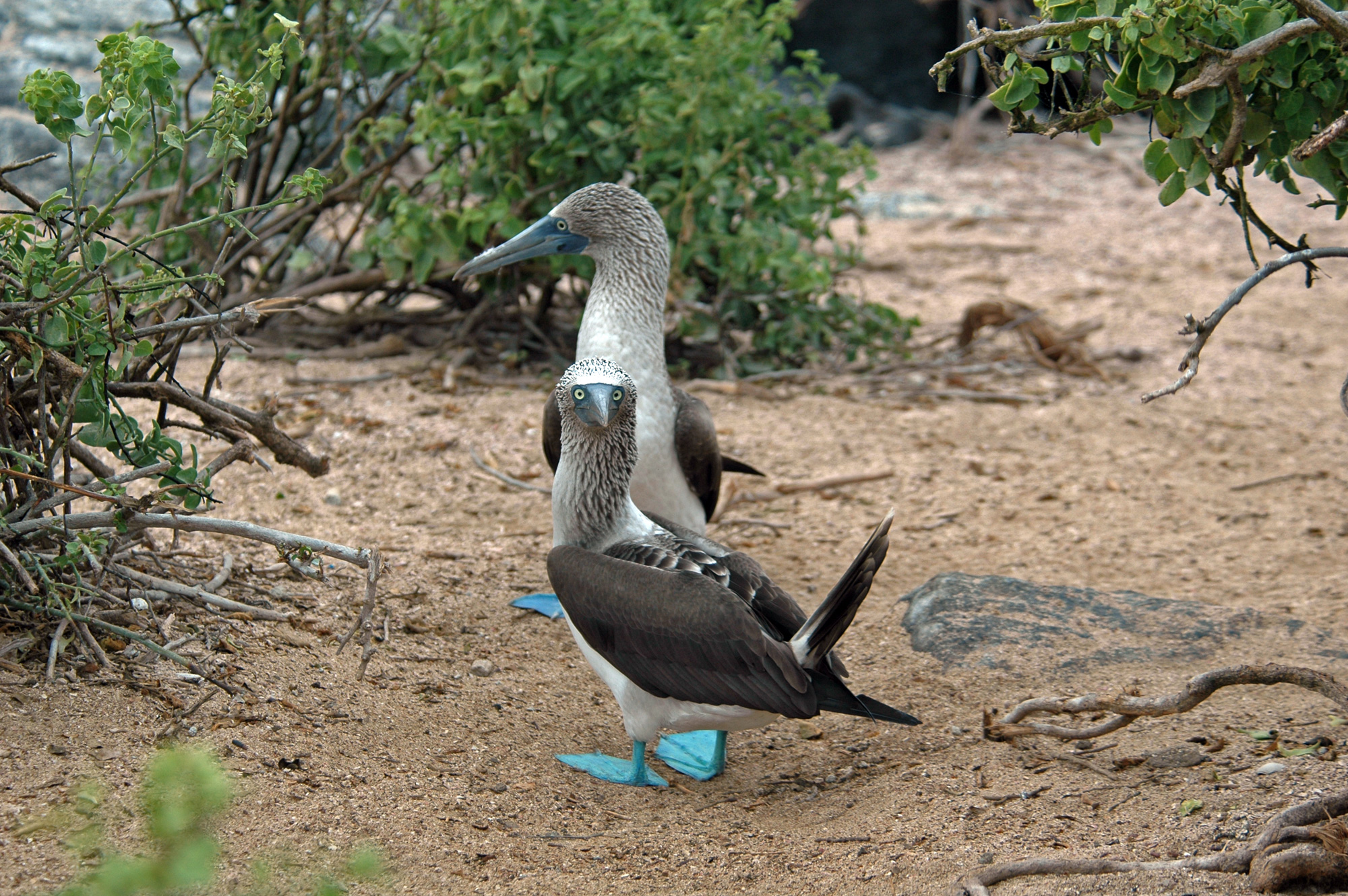This photograph captures two birds standing on a desert-like, sandy ground punctuated sparsely with small bushes, rocks, and dead branches. Both birds are notable for their bright turquoise blue feet and brown wings with brown tails. Their breasts are distinctly white, while their necks and the tops of their heads display varying shades of brown and white. The beaks are a dark green-blue color and appear fairly long. The bird in the foreground is smaller and faces the camera directly, with its tail extended straight up, suggesting it may be a chick. Its wings are dark gray, and its back features gray and white speckles. The larger bird behind it has a seemingly longer beak and neck, which is predominantly white. Both birds have beady eyes and are similarly colored. The terrain around them is mainly sandy and grainy, representative of a desert habitat.